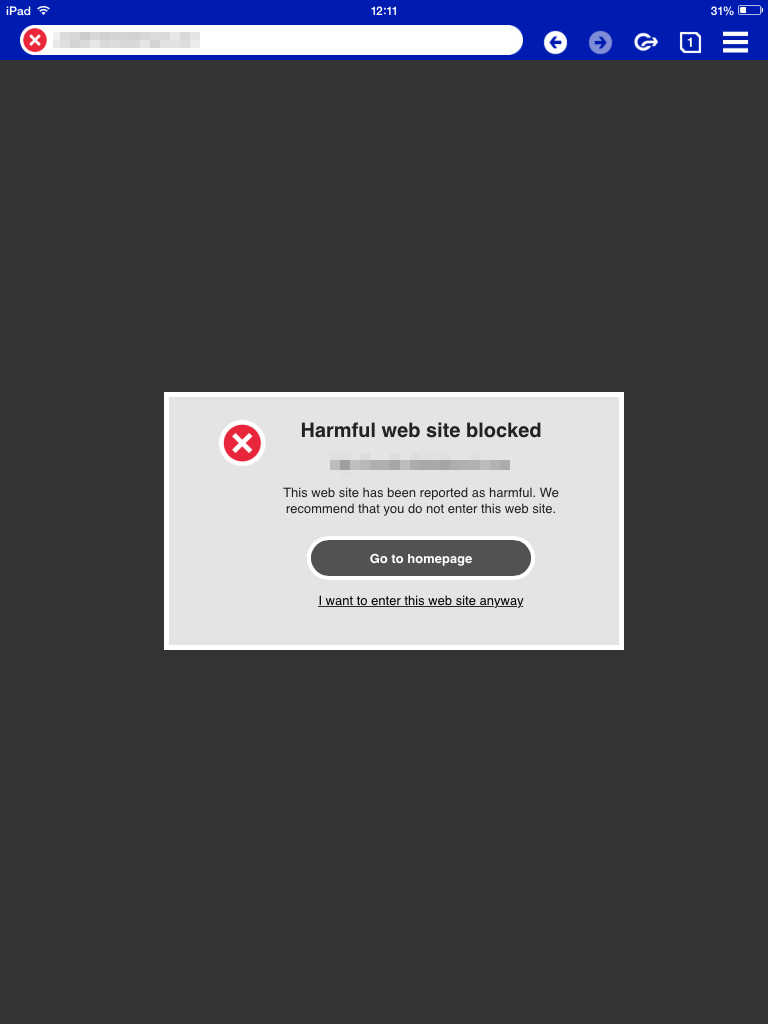In the image, a basic page from an iPad screen is displayed prominently. The top left corner displays the text "iPad," confirming the device type. The status bar at the top indicates the current time as 12:11 p.m. and shows a low battery level at 31%. The screen is displaying a web page with the address bar intentionally blurred out to obscure the website's name. Next to the blurred address bar is a red "X" icon, accompanied by the standard back and forward navigation buttons.

The browser appears to have only one open tab. Dominating the screen is a warning message that reads "Harmful website blocked." Below this header, it states, "This website has been reported as harmful. We recommend that you do not enter this website." There is a button labeled "Go to Home Page," and below this button is a link that says, "I want to enter this website anyway," which is underlined for emphasis. The background of the screen is a dark gray, giving a somber tone to the warning. The image primarily conveys a security alert on the iPad, advising the user against visiting a potentially harmful website.